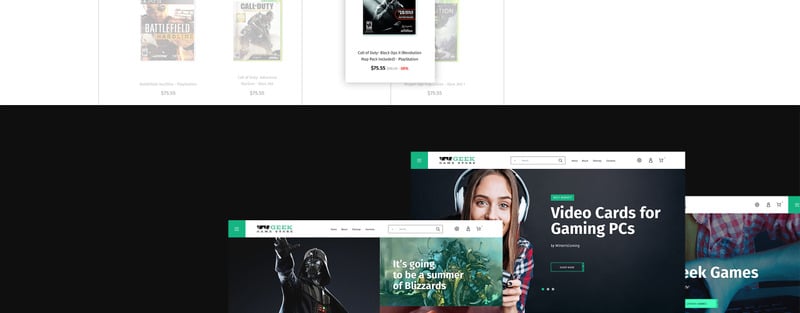The image features a vibrant and eclectic collage centered around various gaming and pop culture themes. Dominantly displayed are titles like "Battlefield," "Call of Duty," with sub-series "Battlefield Hardline" and "Call of Duty: Black Ops." In the middle of the board, there is a conspicuous black section with white text that reads "Geek." The collage also includes a notable image of Darth Vader, symbolizing a strong connection to the Star Wars franchise, and another image suggesting a similarity to Blizzard's tentacled creature designs.

Additional elements on the board include a set of headphones, indicating an auditory element or potential gaming accessory, and a depiction of a person with brown hair. Text related to "video cards for gaming PCs" suggests a focus on high-performance gaming hardware. The overarching theme of the collage appears to lean heavily on gaming, as shown by the scattered text such as "Geek Games," and various visual templates or snapshots that may represent different gaming genres or digital interfaces. White text overlays are seen throughout, adding to the layered complexity of the image.